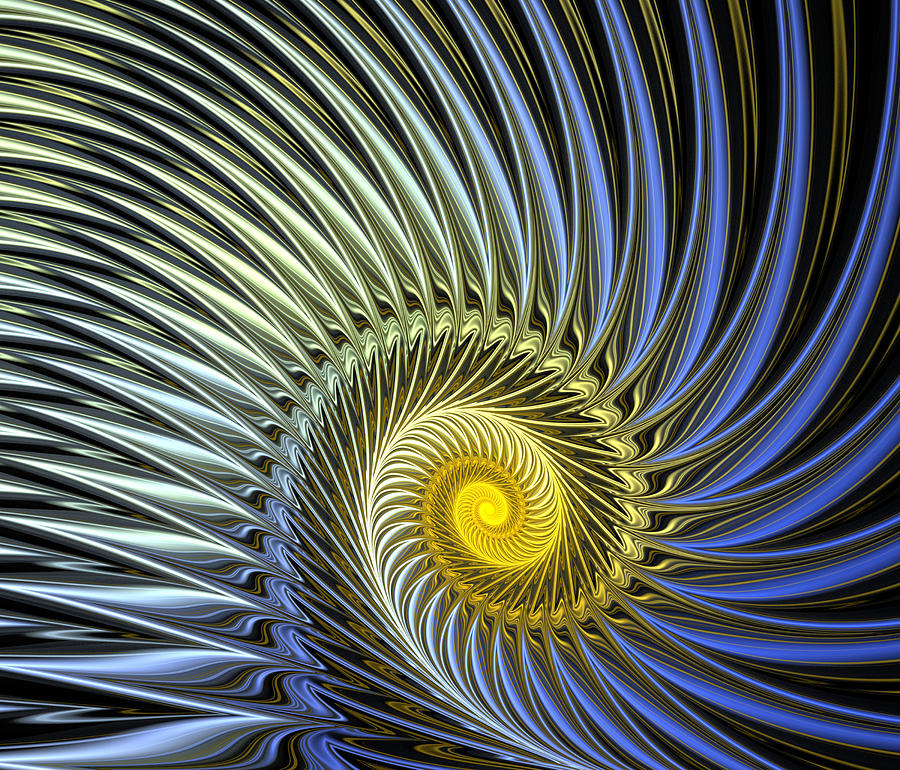The image appears to be a highly detailed, abstract design rendering, possibly created by artificial intelligence or inspired by a mathematical equation. It features a prominent spiral movement that winds inward towards the right, becoming progressively tighter towards the center. The spiral consists of wavy, feathered spokes that give off a metallic and shiny appearance. The outer edges of these spokes are predominantly blue and white, with some streaks of beige and silver, resembling bird feathers that fan out. As the spiral tightens, the colors transition to more silver and black before leading to a bright, glowing yellow center. The composition lacks any discernible background or text, emphasizing the intricate, high-definition 3D art form. Ultimately, the image evokes a sophisticated and dynamic aesthetic, reminiscent of something found in a design book.